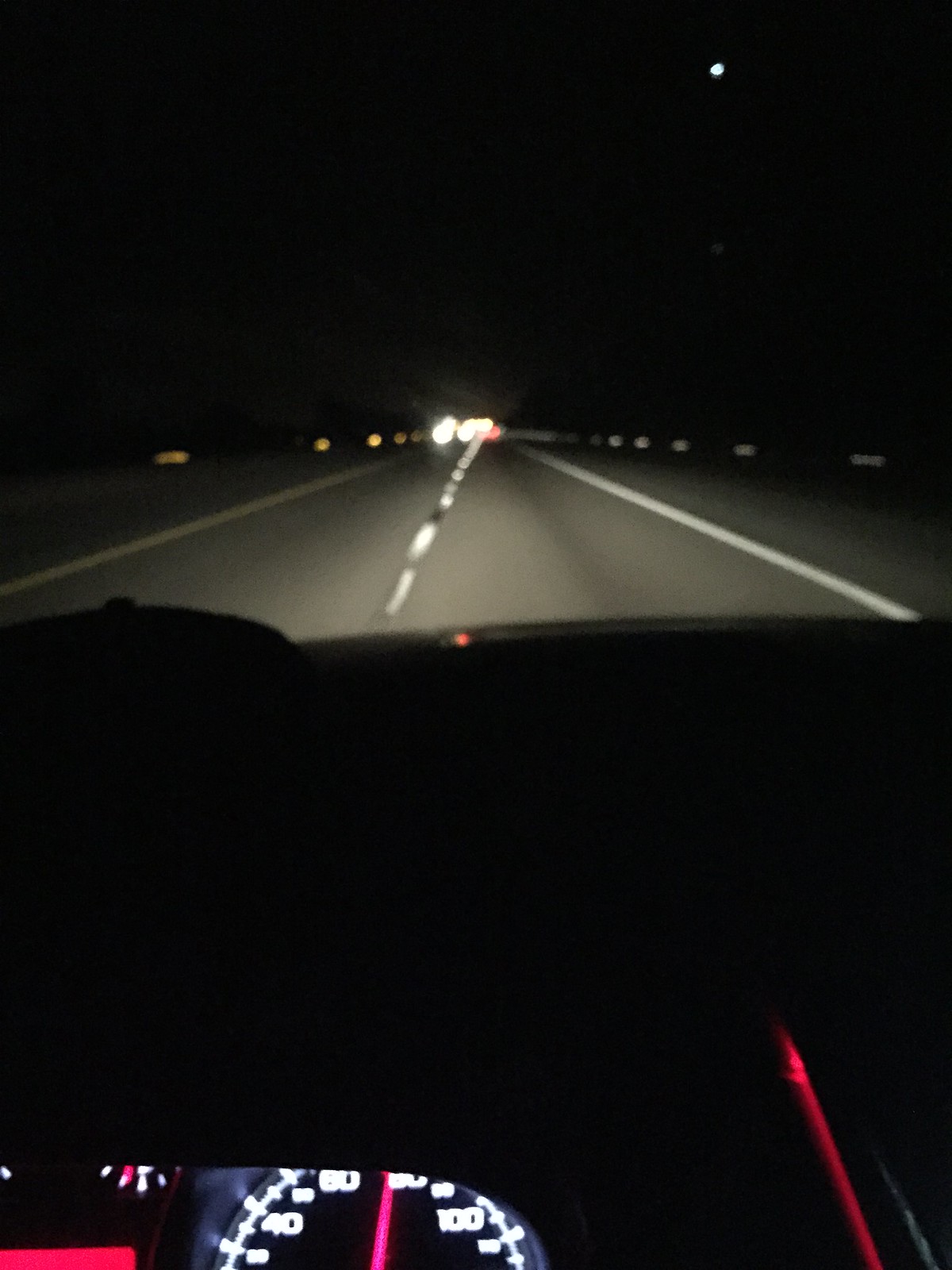A night-time photograph taken from the driver's seat of a car captures a vertical rectangle view through the windshield. The illuminated dashboard is prominently featured, with a partial view of the speedometer showing the red needle hovering near the 80 mark. The numbers are clearly visible but appear slightly too bright and somewhat blurry. The top portion of the dashboard fades into complete darkness. The concrete road ahead is faintly lit, marked by spaced white lines and bordered on the right by continuous white road lines. Distant car headlights are visible, creating a glowing effect that diffuses outward. Scattered throughout the background are small, indistinct light dots, with a noticeable single white dot high in the black sky, possibly a distant star or a distant streetlight.